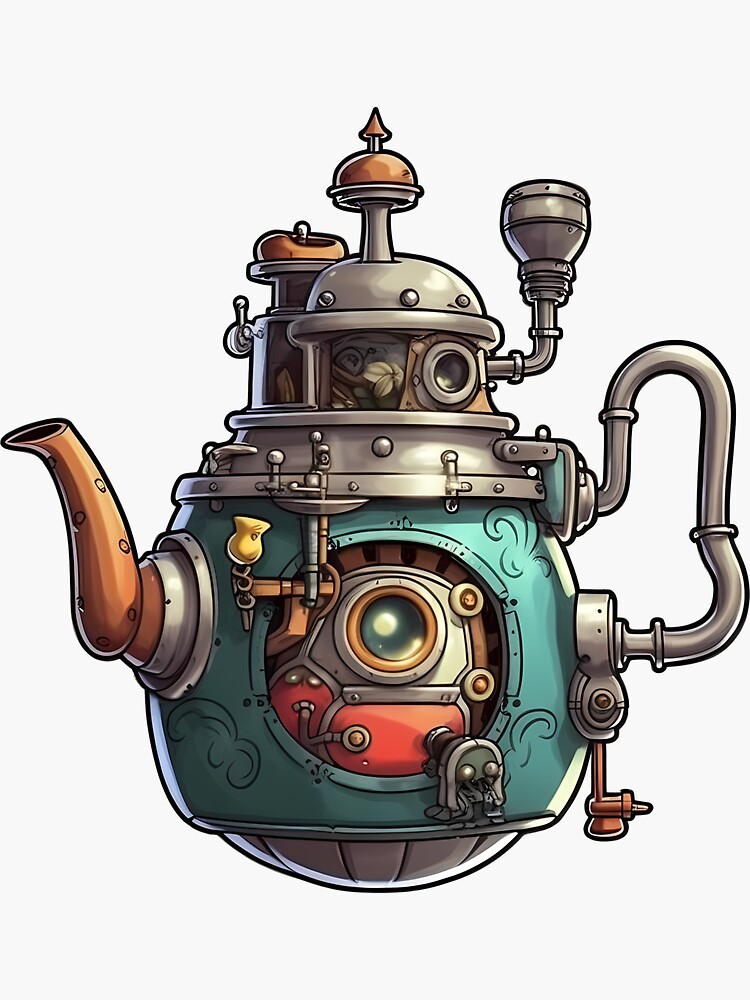This whimsical drawing, possibly rendered in colored pencil or watercolors, showcases a steampunk-style teapot with submarine elements, likely created digitally. The teapot's teal-colored body features intricate brass and silver accents. A brass spout protrudes from the left side, while a silver, pipe-like handle extends from the right. Dominating the center of the teapot is a large, circular glass lens, resembling a pressure window or possibly an eye, suggesting the teapot may also serve as a vessel for an occupant. The top of the teapot features a bronze, bell-shaped structure with an additional circular eye-like element, surrounded by tubes and pipes, creating a hatch-like appearance. Completing the steampunk aesthetic, a propeller is attached to the bottom right, further enhancing the submarine impression.